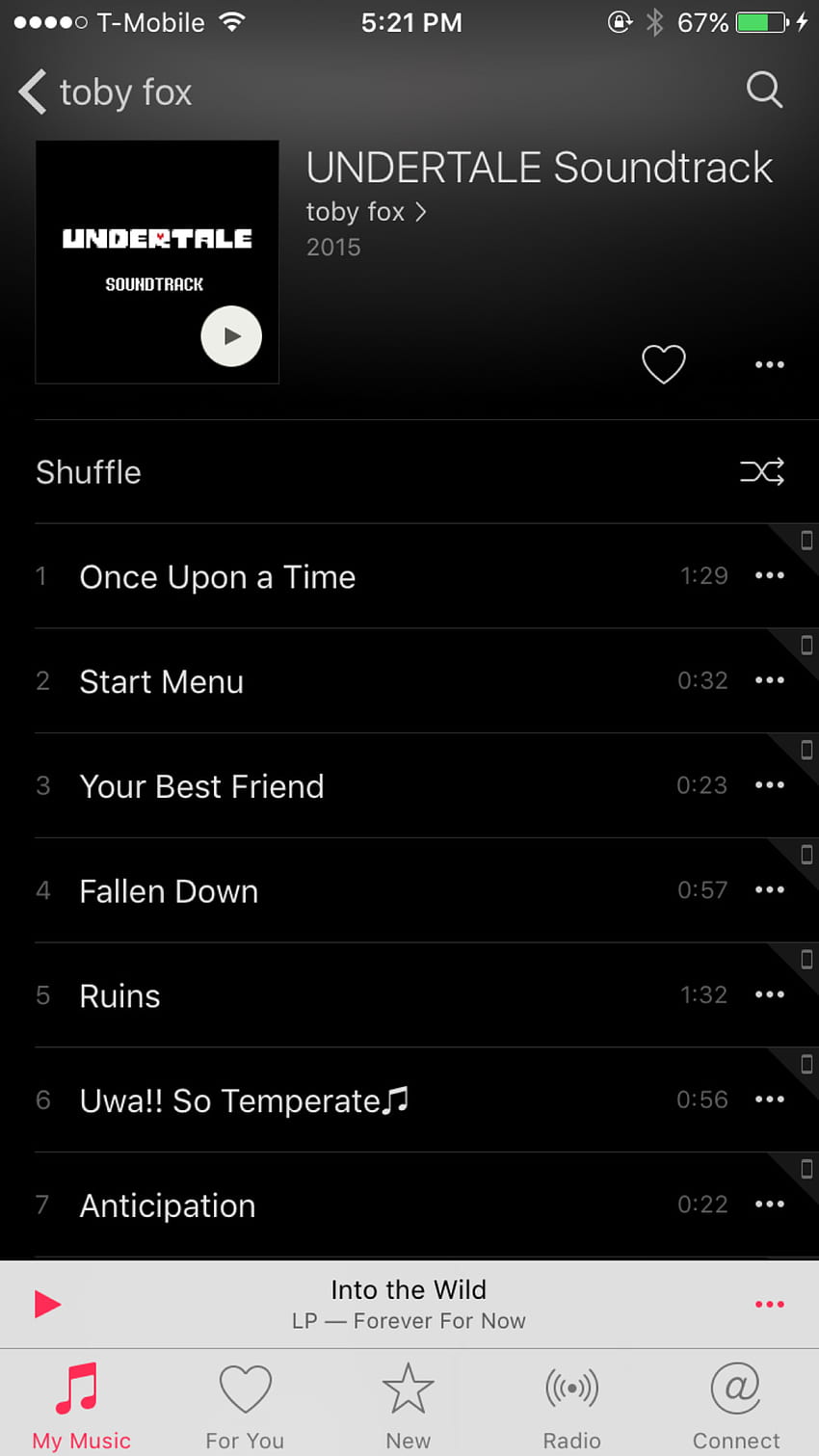This image captures a screenshot of a mobile device's interface. Starting at the top left corner, the network signal strength is displayed with 4 out of 5 bars, followed by the T-Mobile network provider name. To its right, the WiFi signal icon shows a full 3 out of 3 bars. Centered at the top is the current time, 5:21 PM. On the far right, several icons are visible: the screen orientation lock, Bluetooth symbol, and the battery indicator showing 67% with the phone actively charging.

Beneath these status icons, text indicates that music by Toby Fox from the "Undertale" soundtrack, a 2015 album, is currently playing. The song list from the album includes titles such as "Once Upon A Time," "Start Menu," "Your Best Friend," "Falling Down," "Rains," "Oh Wa," "So Temperate," and "Anticipation." The song currently playing is "Into The Wild." Additional album titles and songs such as "LP" and "Forever For Now" are also mentioned.

At the bottom of the screen, navigation categories include "My Music," "For You," "New," "Radio," and "Connect."